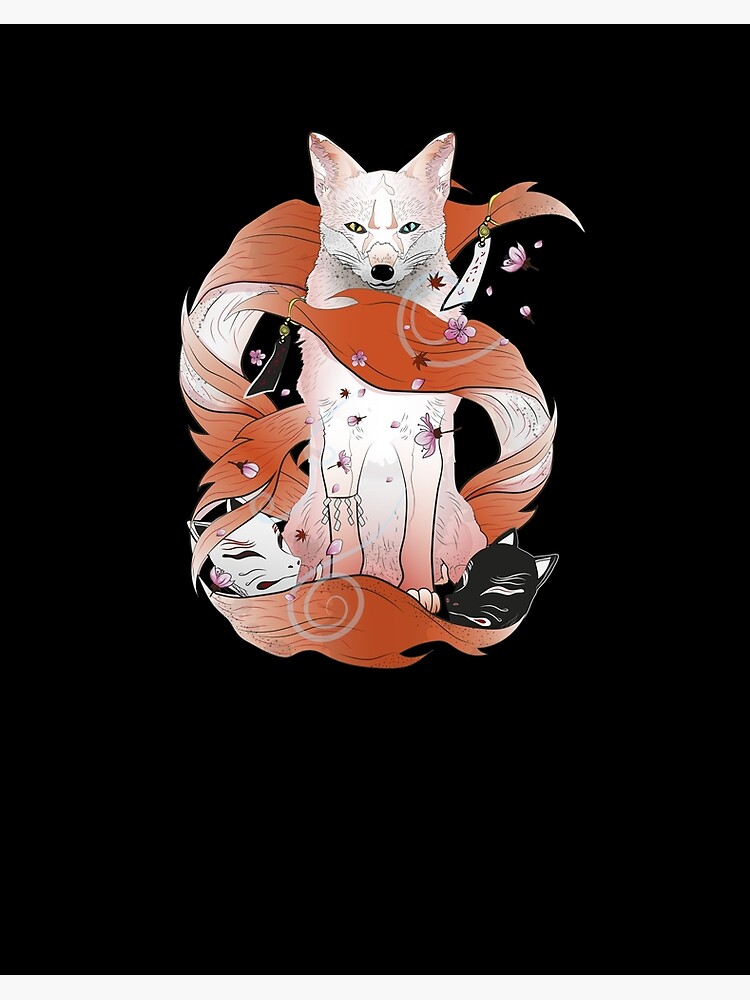The image is a detailed painting of a fox-like creature set against an entirely black background in a portrait layout. The focal point is a predominantly white fox with hues of pink, orange, and light brown accentuating its fur. The fox, sitting with its front legs up and its hindquarters on the ground, stares directly at the viewer with two differently colored eyes—one yellow and one blue. It also features black whiskers, a black nose, and a small black mouth.

The fox has an unusually long tail that coils around its body in multiple sections. Portions of the tail are coral-colored while others remain white. One segment wraps around the fox's neck, another covers its chest, and yet another drapes over its feet. Scattered around this intricate tail are delicate purple flowers, adding to the painting's visual complexity.

Attached to the tail are two tags: a white tag hanging from the top and a black tag from the middle, each secured with a green clasp. At the base of the fox's tail on either side are two fox masks—one white with pink details and one black with white outlines—facing each other. The combination of these elements creates a mesmerizing and mystical portrayal of the fox, elevated by the stark contrast of the black background.